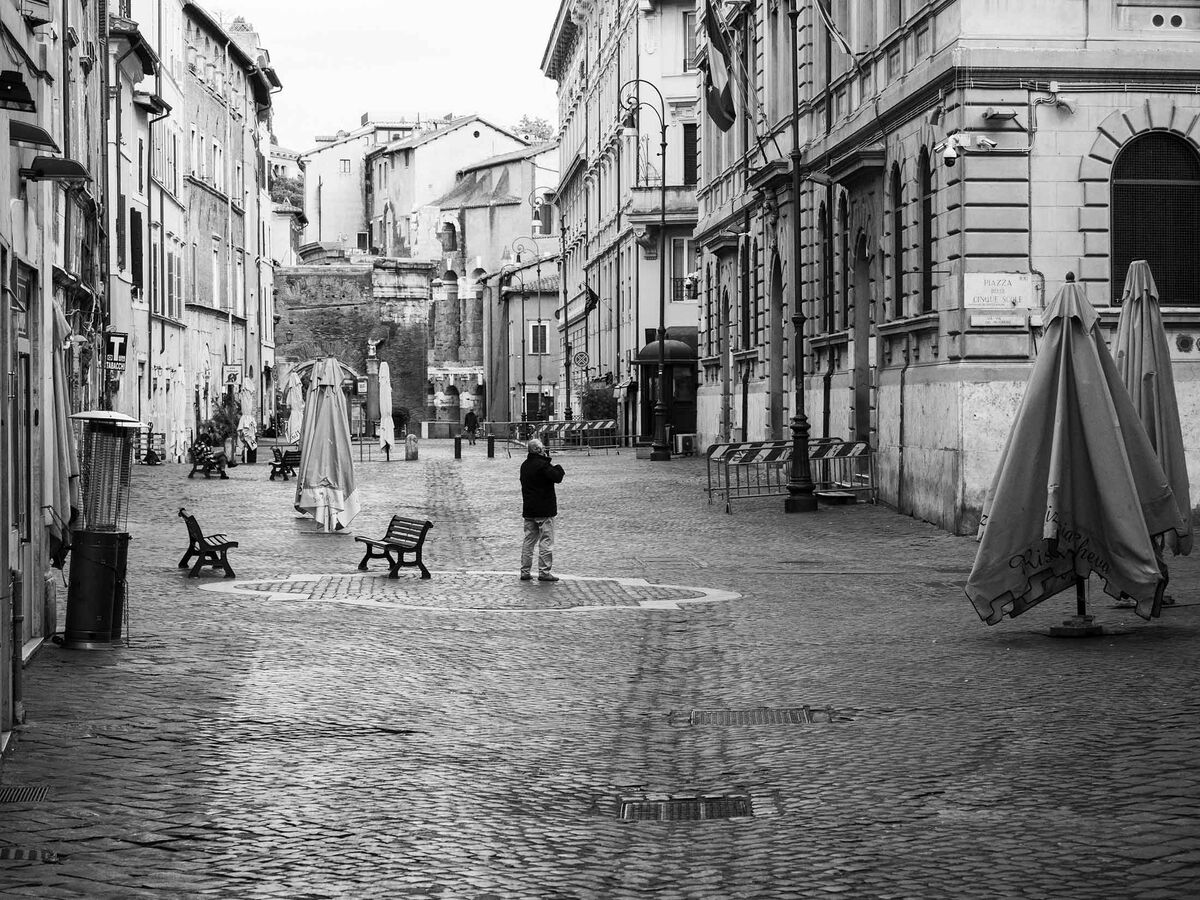This black-and-white photograph captures a detailed, ground-level view of a Western European urban alleyway framed between rows of old-fashioned masonry buildings with ornate stone decoration and arched windows. The cobblestone street features a central ditch with a visible grate, and a second grate slightly above and to the right. In the foreground, there is a small marked area where an older gentleman stands with his back to the camera, wearing a black jacket and beige pants. His arms are positioned in front of him as if he's holding something. To his left are two benches facing each other, and beside them, a trash can. The alleyway is bordered by several stone buildings, and scattered throughout are black lampposts and multiple tall closed umbrellas, adding to the charm of the scene. In the background, the alley slopes upward slightly, with additional buildings visible in the distance, creating a sense of depth and crowded architectural beauty. Despite the urban density, the street itself appears largely unoccupied, save for the lone man, enhancing the vintage and serene atmosphere of the photograph.